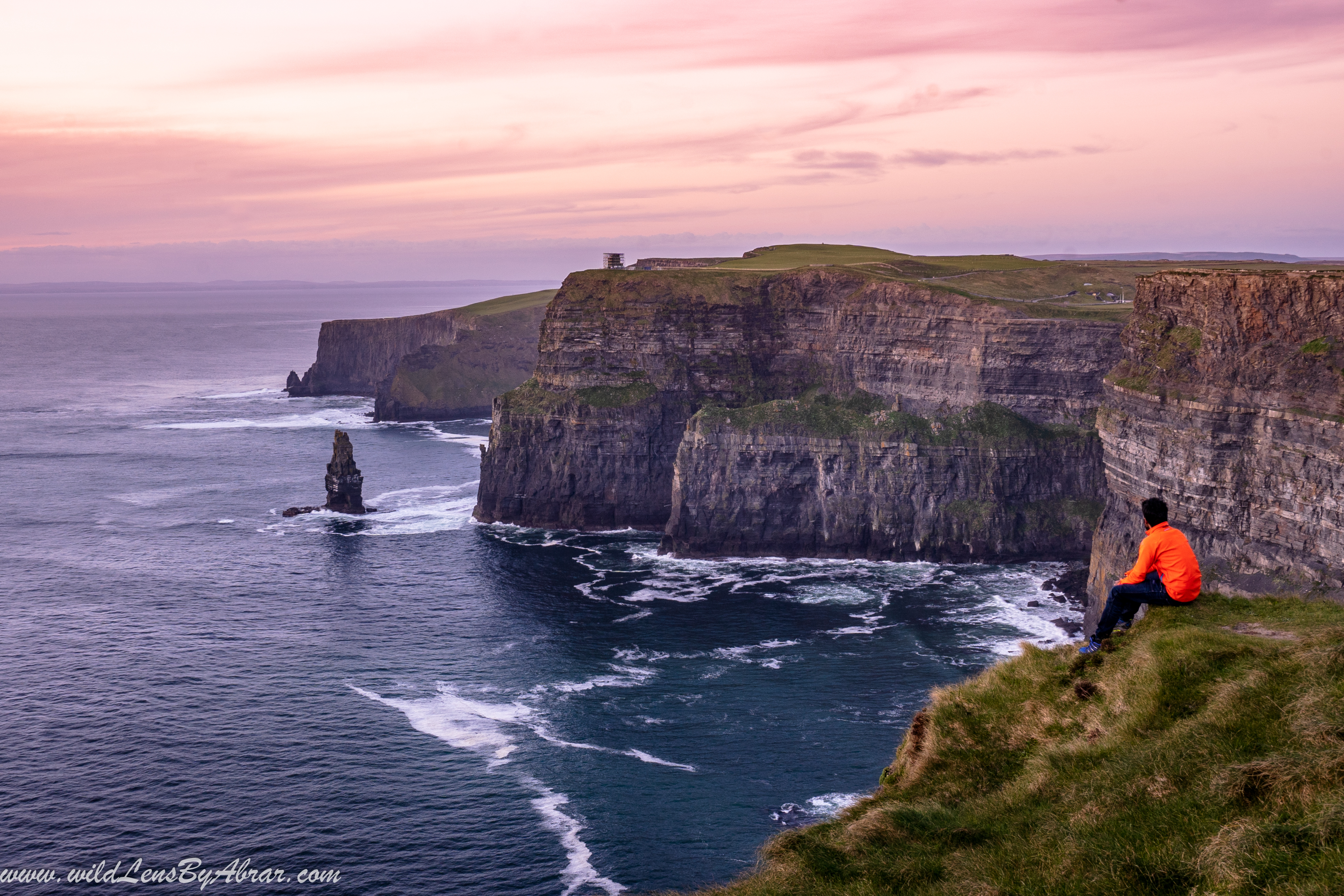In this stunning full-color outdoor photograph, captured by natural light at what appears to be sunset, we see an expansive, horizontally rectangular view of dramatic coastal cliffs. In the lower right corner, a man dressed in jeans and a bright orange jacket sits on the grassy edge of a bluff, gazing out over the striking scenery. The cliffs, some featuring sharp, tall rock formations, cascade steeply downwards into the vivid blue ocean, which turns frothy white where waves crash against the rugged rocks. The sky above is painted with soft pink hues and dotted with scattered clouds, enhancing the tranquil yet awe-inspiring atmosphere of the scene. In the lower left corner, subtle text reads "www.wildlensbyabrar.com," attributing the image to its creator. The entire scene evokes a sense of majestic natural beauty, with no barriers between the serene grassy tops and the sheer, plunging drops below, suggesting a wild and untamed landscape that might resemble the coasts of Scotland.